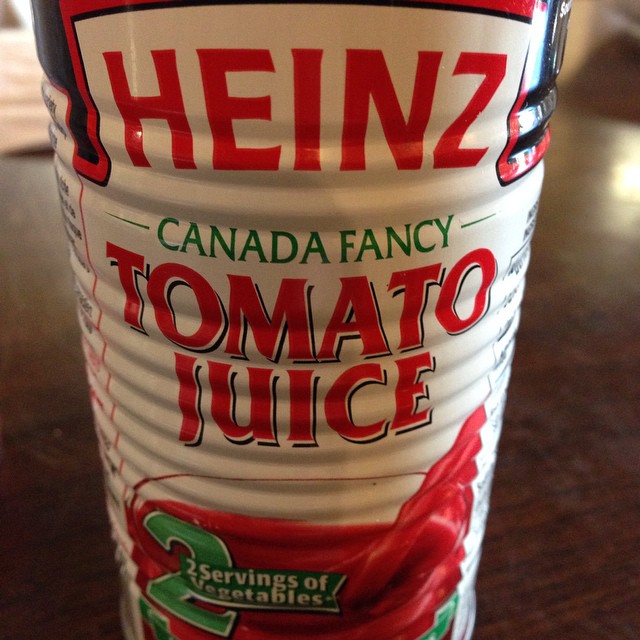The image depicts a close-up of a Heinz tomato juice can resting on a brown wooden table. The can features horizontal ribbing along its sides. The label predominantly displays a white background with various text and graphics. At the top, the word "Heinz" is prominently printed in large, red, capital letters. Below this, "Canada Fancy" is written in green text with horizontal green lines flanking the 'C' and 'Y.' Following that, "Tomato Juice" is boldly presented in red text with a black drop shadow. A glass filled with tomato juice, and possibly a red utensil sticking out, is illustrated beneath the text. Over the image of the juice, a green rectangular banner states "2 servings of vegetables" in white letters.